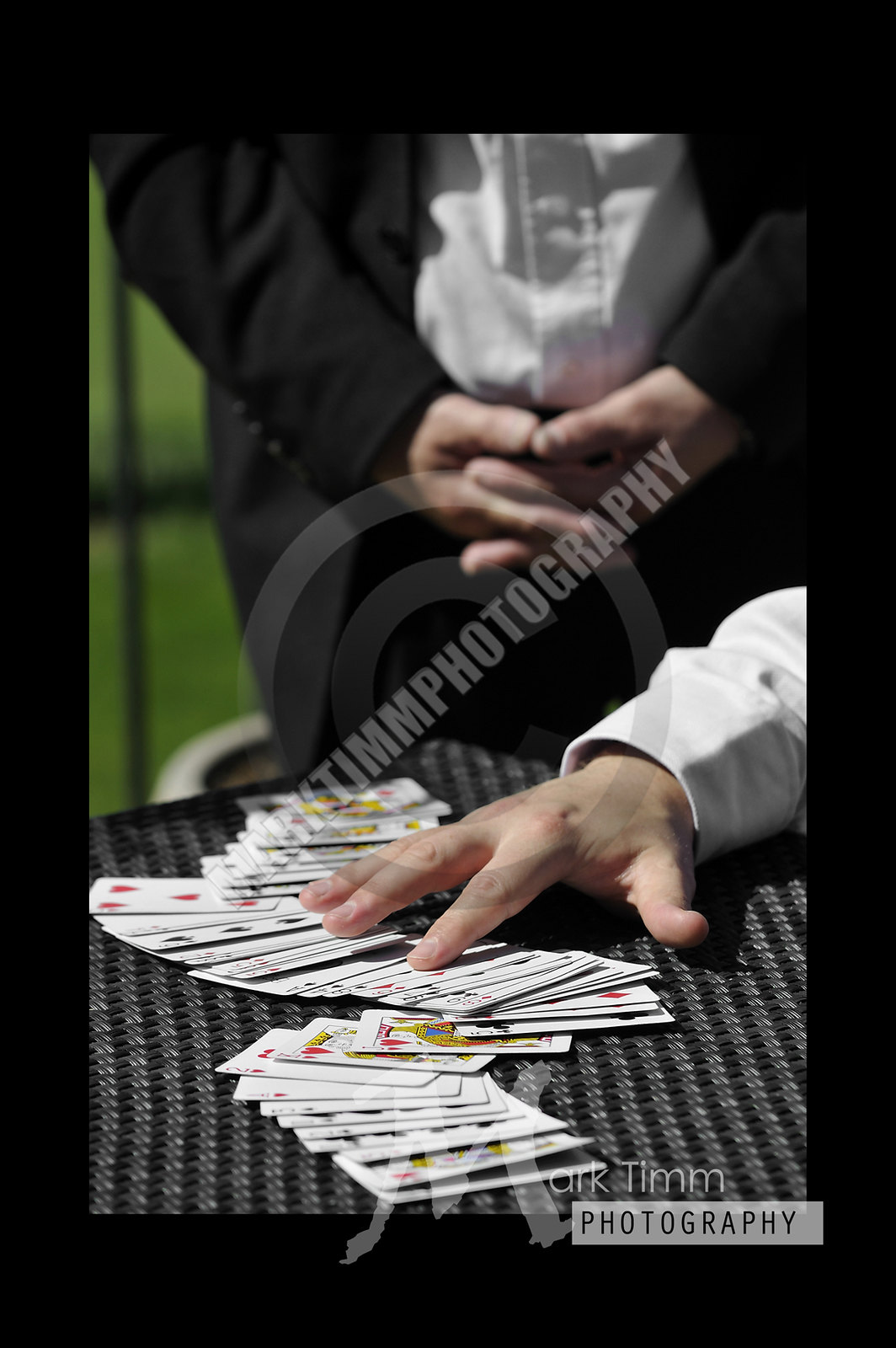This photograph, captured to promote Arc Timm Photography, presents a dynamic scene centered around a game of cards. In the foreground, a man dressed in a crisp white shirt is visible from the shoulder down. His arm extends forward, his hand resting on a table covered with a spread of playing cards, all facing up. One of his fingers is lightly touching a card, suggesting a moment of decision or contemplation.

Accompanying him in the background is another man dressed formally in a suit jacket, slacks, and a white shirt, sans tie, standing with his hands folded in front of him. This second individual provides a composed and observational presence as he overlooks the scene.

The setting is a table draped in a predominantly black tablecloth, detailed with a pattern of interlinked white zeros forming a continuous line. The backdrop of the photograph includes a window on the left side, framed with black molding. Through the window, the hint of greenery outside suggests a peaceful environment with a lawn or bushes.

At the bottom of the image, a watermark reads "Arc Timm Photography," lending a professional and artistic touch to the composition. The scene is thoughtfully arranged, offering an intriguing blend of action and ambiance.